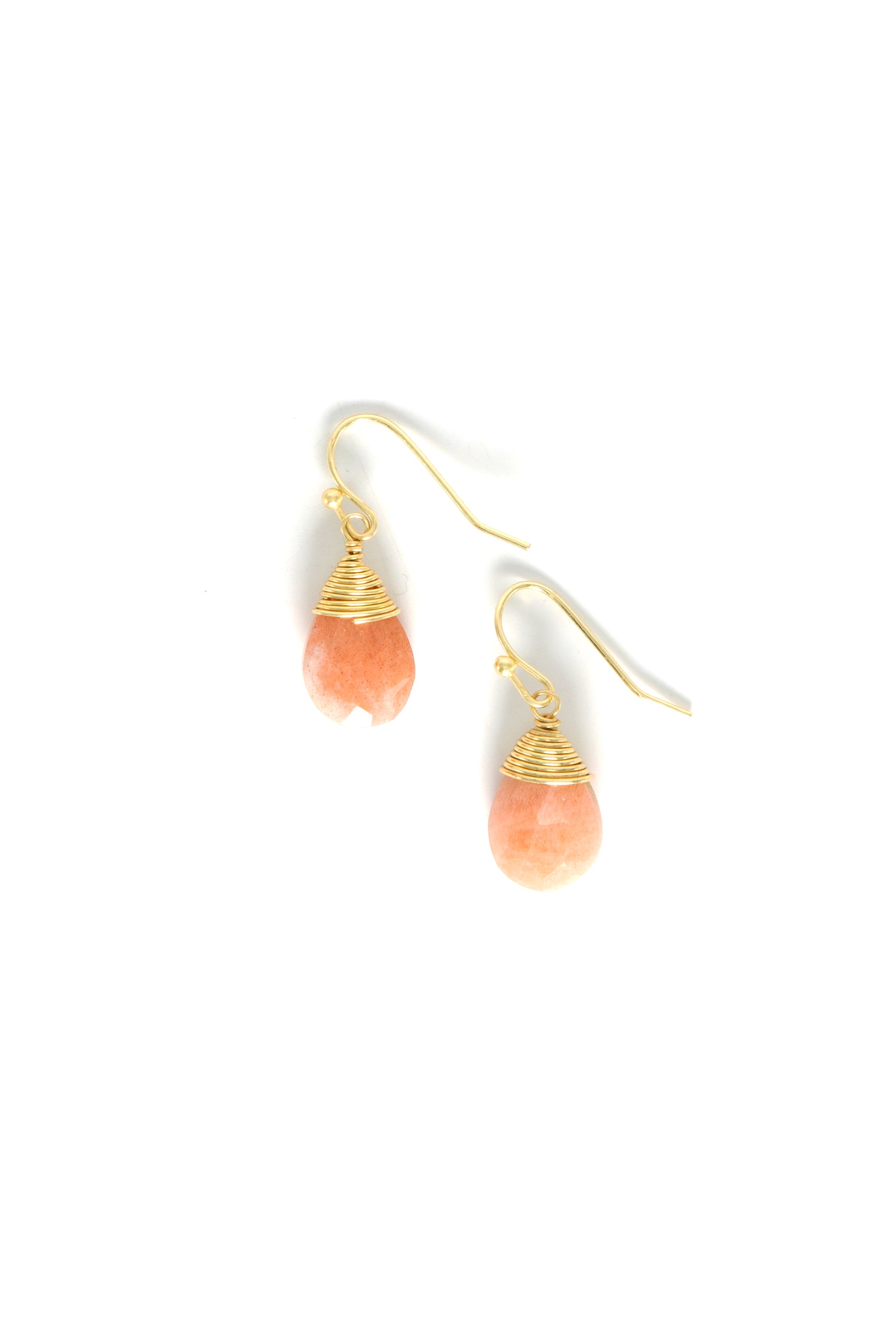The image showcases a pair of delicate, light salmon-pink, teardrop-shaped gemstone earrings on a stark white, overexposed background. These dangle earrings are designed for pierced ears, with each stone meticulously wrapped at the top with gold wire, creating a secure and ornate loop that connects to gold fish hook-style earring hooks. The gemstones, likely Pink Chalcedony, have white and coral-like inclusions adding to their intricate appearance. The earrings, which cast subtle shadows on the bright background, appear small and lightweight but prominently feature the sizable, faceted stones, adding an element of elegance and charm.